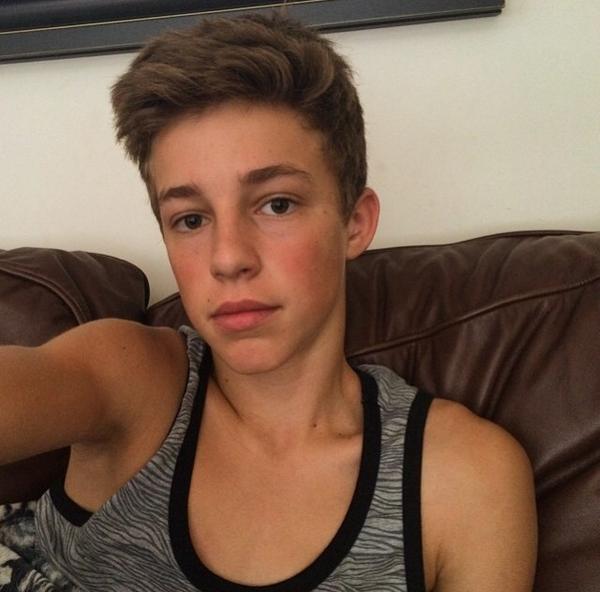In the photograph, a teenage boy, likely around 14 or 15 years old, is taking a selfie. He is seated on a brown leather couch in front of a cream or light-colored wall. Notably, a black-framed picture hangs just above his head. The boy, who has a reddish tan complexion, features short, dark brown hair that is slightly longer on top and closely cut on the sides. He has dark brown eyes, brown eyebrows, and somewhat rosy cheeks. His build is slim, accentuated by prominent collarbones visible due to the light gray tank top he is wearing, which has a small zebra print design with black outlining around the collar and armholes. His extended left arm suggests he is holding a phone towards himself to capture the snapshot.